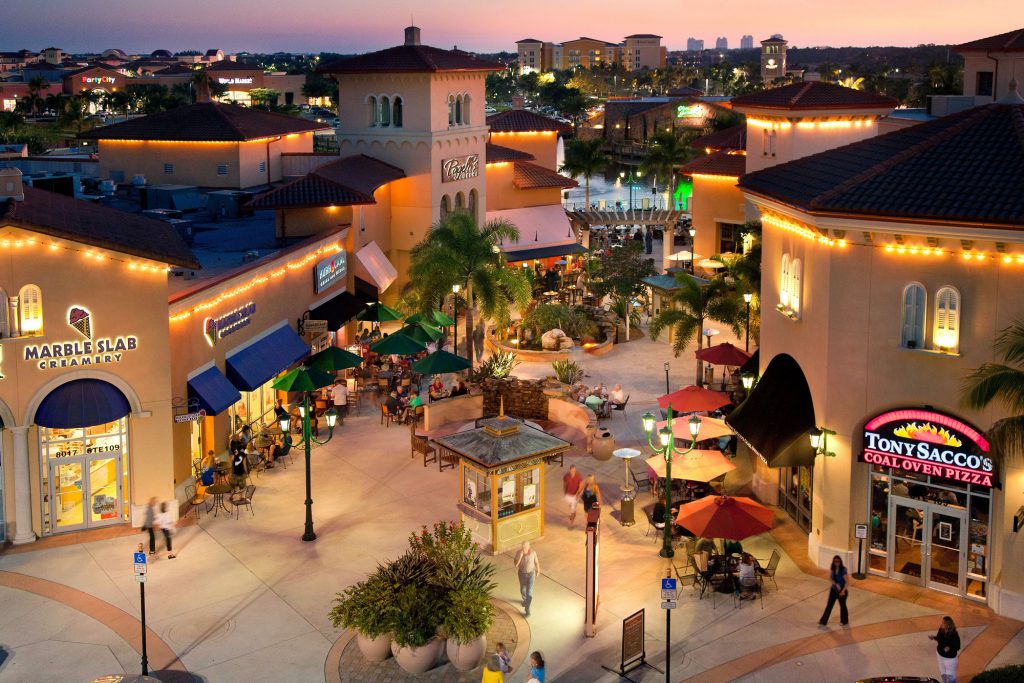The image captures a dynamic, slightly aerial view of an outdoor shopping plaza just as evening approaches, with a sky transitioning from pink to dark gray-blue. The plaza, bustling with tourists and locals, features well-lit beige and brown buildings such as Tony Sacco's Coal Oven Pizza on the right and Marble Slab Creamery on the left. The scene is rich with detail, showcasing tiled pavements, street lights, and various stores adorned with blue, white, and black awnings. Red and yellow umbrellas mark a nearby cafe, while potted plants and palm trees add a touch of greenery amidst the robust downtown area.